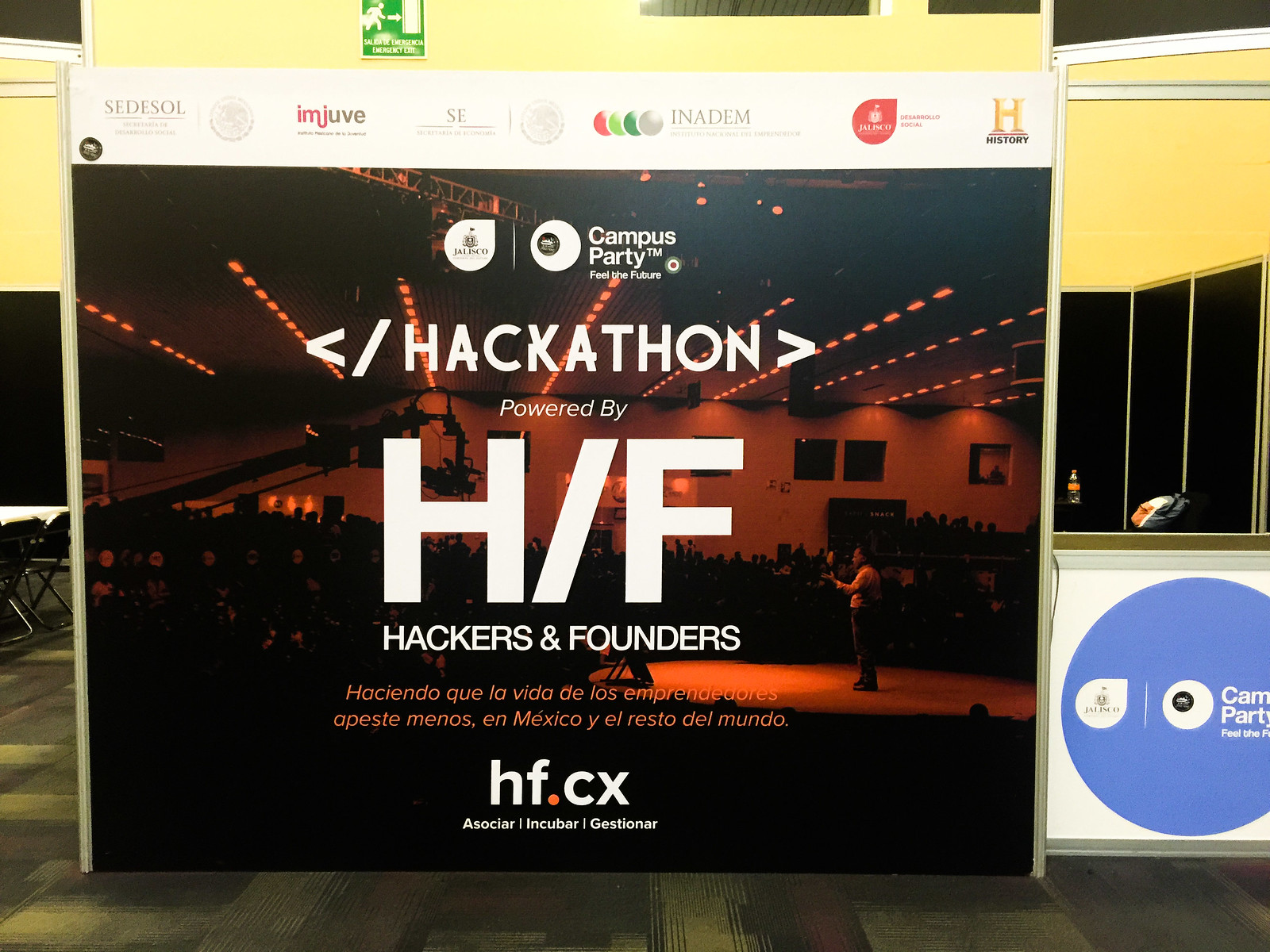The image depicts a large, square-shaped poster set against a yellow wall, with part of a grays and greens toned carpet visible below, indicative of a convention center setting. Leaning against the left side, there are some folding chairs. On the bottom right of the image, there is a small white sign featuring a blue circle design. The poster itself includes a vivid, red-filtered photograph of a speaker addressing a crowd, with a camera boom cutting through the scene. The top section of the poster is adorned with logos for various entities, including Setasol (S-E-D-E-S-O-L), Juve (I-M-J-I-M-J-U-V-E), and the History Channel. The main text overlaying the image reads in white: "Campus Party Feel the Future Hackathon powered by H/F hackers and founders." Below, there is Spanish text: "haciendo que la vida de los emprendedores apeste menos en México y el resto del mundo" and "asociar, incubar, gestionar," followed by the URL "hf.cx".